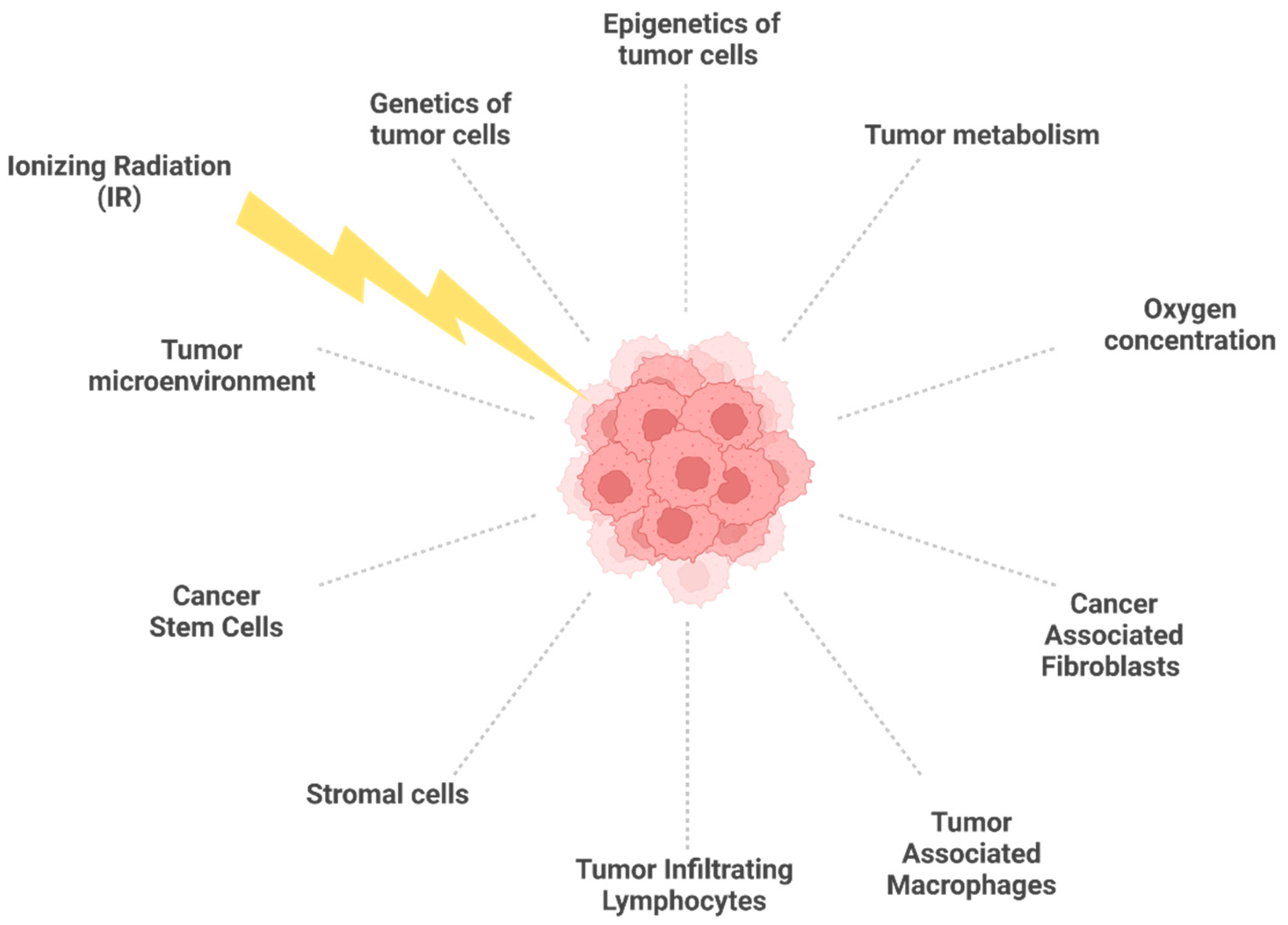The image depicts a medical poster or chart on a solid white background. At the center of the chart is a pink mass consisting of about ten different pink blobs or balls, arranged in a way that they almost resemble a flower or a pine cone. This central pink formation represents tumor cells. Around the central pink mass, like the numbers on a clock, are various terms and statements linked by dotted black lines, with each term describing different aspects or influences on the tumor cells. Starting from the top at the 12 o’clock position and moving clockwise, the terms are: 'Epigenetics of tumor cells', 'Tumor metabolism', 'Oxygen concentration', 'Cancer-associated fibroblasts', 'Tumor-associated macrophages', 'Tumor-infiltrating lymphocytes', 'Stromal cells', 'Cancer stem cells', 'Tumor microenvironment', 'Ionizing radiation'—which is connected to the central pink mass with a lightning bolt rather than a dotted line—and finally, 'Genetics of tumor cells'.